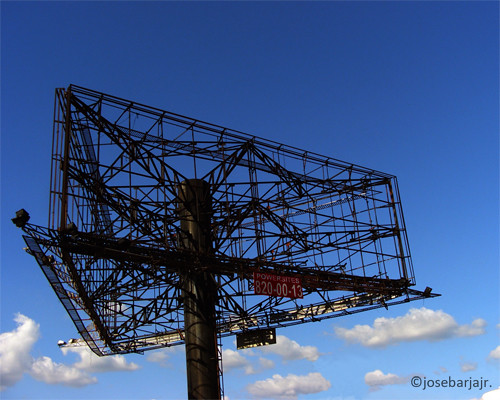This vivid color photograph offers an up-close view of a sophisticated antenna or receiver set against a stunningly vibrant blue sky. The majority of the composition is dominated by an intricate, large, dark wire structure, likely black, which features a prominent vertical pole intersected by a cross beam. The design includes a complex mesh that forms a distinctive triangle-like shape. Bright and beautiful, the sky fills the background, with lighter blue hues and a scattering of soft clouds adorning the lower portion of the image. In the lower right-hand corner, a copyright symbol is visible alongside the name "Jose Barjajr."